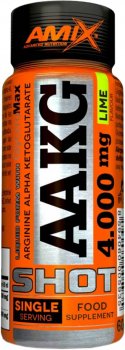This image depicts a vibrant food supplement bottle primarily in orange with a mix of black, silver, white, and lime-colored accents. Dominating the label, "AAKG" is prominently displayed alongside "Arginine Alpha Ketoglutarate". The bottle provides a dosage of 4,000 milligrams and is flavored with lime, clearly marked in black font against a yellow background. The product is identified as a single serving food supplement, with these words featured at the bottom in silver and orange fonts respectively. The black cap is detailed with ridges and bears the brand name "Amix" in orange, with the "X" distinctly larger and in a different font. Additionally, a partially visible nutrition label wraps around the bottle, although the text remains unreadable. Silver and black lettering also run vertically on the left side of the bottle, ending with the word "Max".